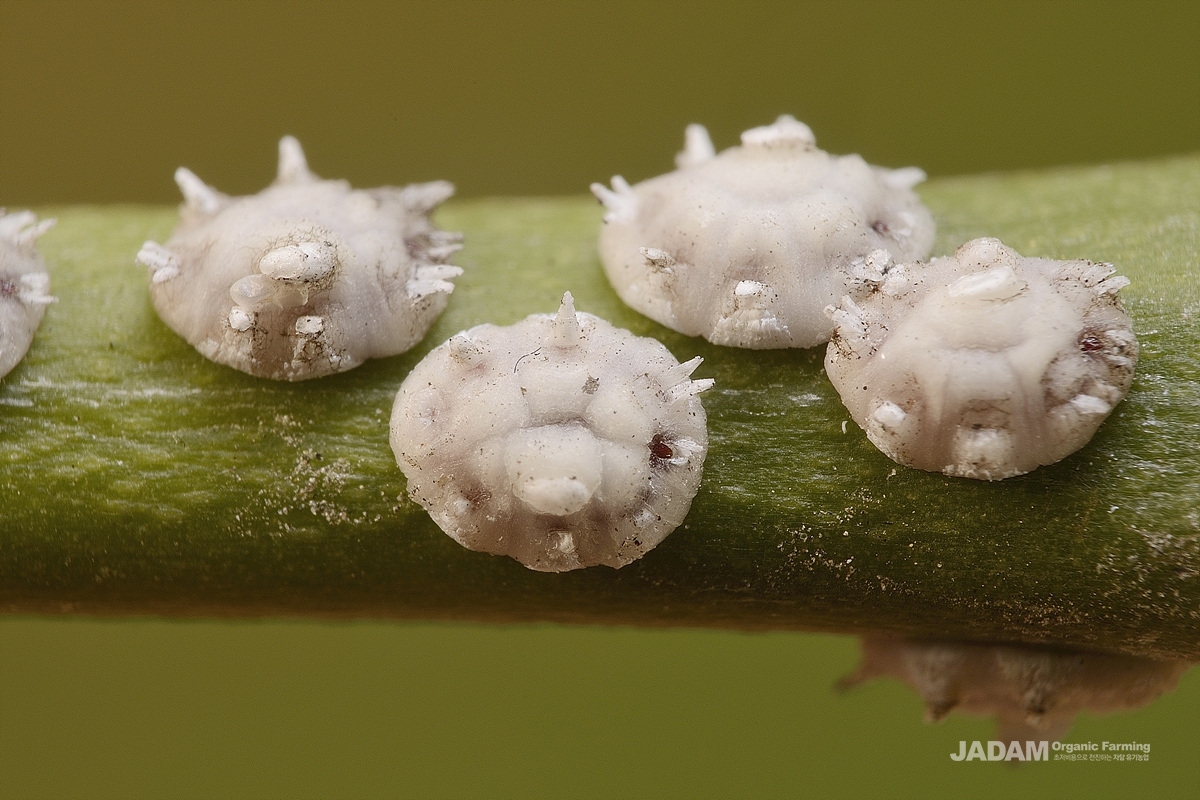This color photograph reveals an extreme close-up of a green plant stem, captured in such detail that it seems almost microscopic. The cross-section of the stem showcases an intriguing array of approximately four small, white, fuzzy growths, which could potentially be mold or fungi. These growths are characterized by their prickly, spiky appearance and seem to cling to various positions on the stem, including one underneath. The background is a gradient of green, darker at the top and lighter at the bottom, providing a blurred, yet complementary setting for the stem. Additionally, scattered brown specks can be seen, adding to the texture and complexity of the image. In the lower right corner, white text reads "JADAM Organic Farming," with smaller Chinese characters beneath it, reflecting the thematic dedication to organic farming techniques.